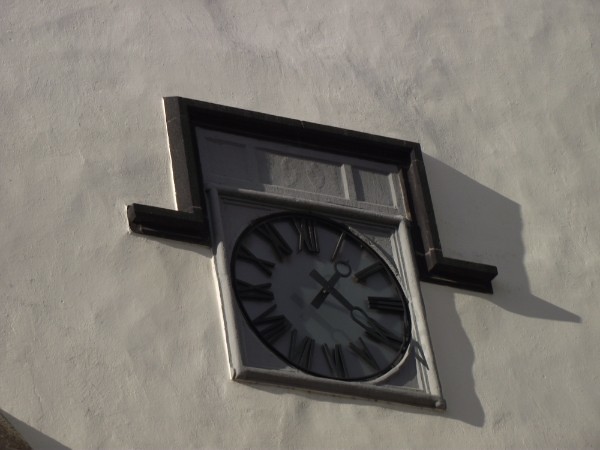In this photograph, we see a detailed, extreme close-up of what appears to be an exterior wall of a building. The wall has a rough, plaster-like texture with numerous shallow ridges, craters, and dents, indicating it might be concrete and is light gray to white in color. Prominently featured in the center of the image is a clock. The clock is housed within a square frame that appears to be made of gray stone. Above the clock, there is a distinctive black rectangular frame or outline shaped somewhat like an inverted and sideways letter 'C' or akin to a square hat resting atop the clock.

The clock itself is constructed from dark iron, reminiscent of 19th-century architectural designs, and features black Roman numerals from I to XII around its face. The clock has two black hands, an hour hand and a minute hand, displaying the time as 1:20. Shadows from the clock and its surrounding structures are cast upon the textured wall, adding depth and dimension to the image.